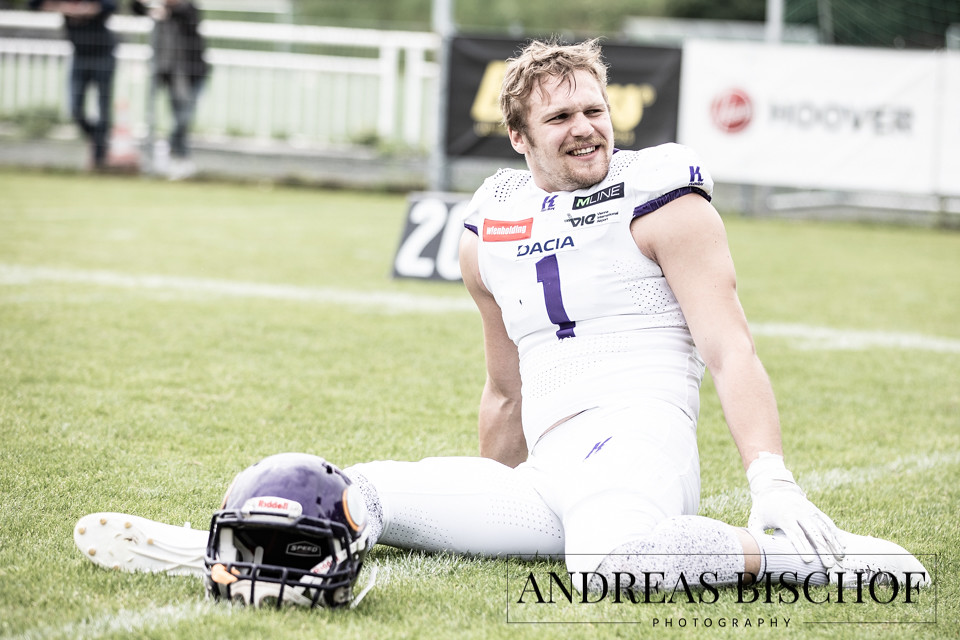The image depicts a close-up, ground-level photograph of a football player on a field, captured by Andreas Bischoff Photography (noted in black text within a see-through rectangle with a black border at the bottom right). The player appears to be in a moment of discomfort, possibly due to an injury. He is sitting on the turf with his right leg extended in front of him and his left leg bent underneath, while grasping his left ankle with his left hand. His face shows signs of pain, with a wrinkled brow. He is fully dressed in white, including his jersey, pants, cleats, gloves, and socks, and sports the number one in purple on his chest, accompanied by advertisements like 'Dacia' and a 'K'. A purple helmet, marked with the Minnesota Vikings logo—featuring a white and yellow-bordered Viking horn—is positioned near him on the green football field, which displays a 20-yard line marker and a banner in the background advertising Hoover. The player, a white man with blonde hair, is the focal point of the image, while the rest of the scene is slightly blurred.